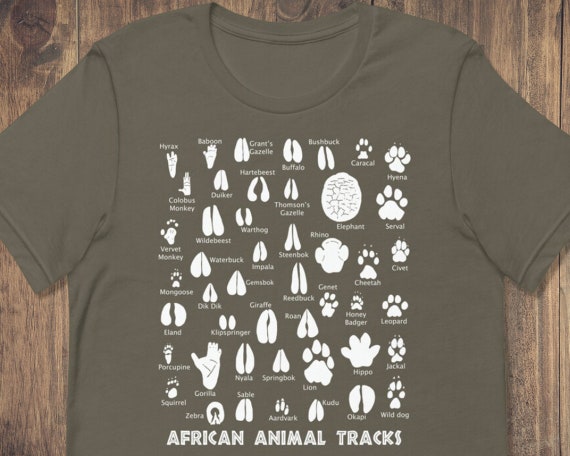The image depicts a t-shirt spread flat against a vertically paneled wooden background. The t-shirt is a dark brown or grey-green color and features an intricate design in white. Covering the shirt are numerous rows of animal footprints, each labeled with the corresponding African animal. Some of the animals listed include Reedbuck, Giraffe, Roan, Leopard, Honey Badger, Porcupine, Hippo, Aardvark, Wild Dog, Jackal, Zebra, Hyena, Elephant, Cheetah, Wildebeest, Baboon, Buffalo, Caracal, Serval, Rhino, Thompson Gazelle, Colobus Monkey, Vervet Monkey, Warthog, Rhino, Steenbock, Zivet, Gemsbok, Squirrel, Gorilla, Sable, Kudu, Okapi, Lion, and Dick Dick, among others. The detailed illustrations and labels make the shirt an informative guide to African animal tracks. At the bottom of the t-shirt, in bold capital letters, it reads "African Animal Tracks."